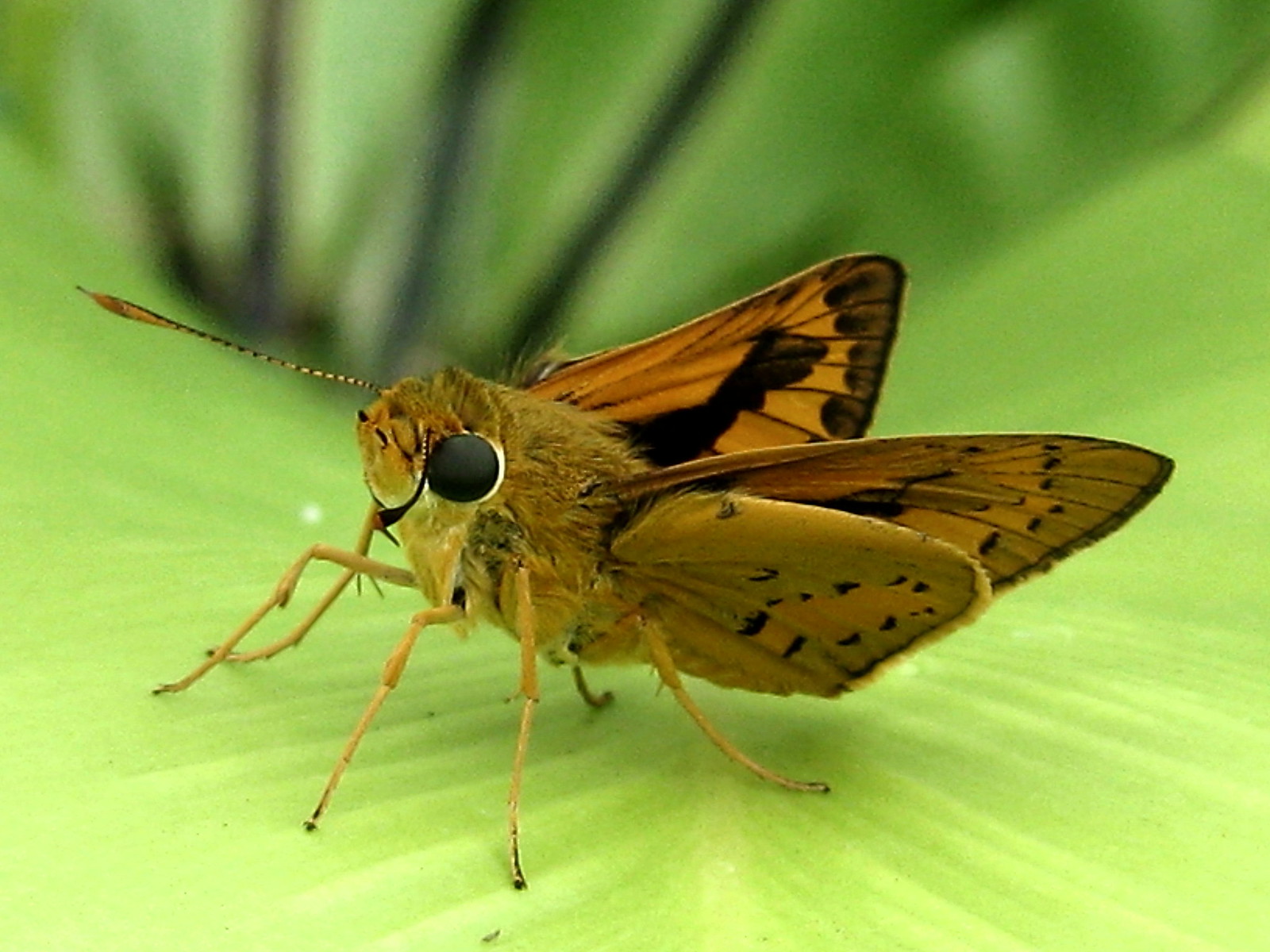The image is a high-quality close-up photograph of a moth perched on a vibrant green leaf, with the background intentionally blurred to keep the focus on the moth's detailed features. The moth, likely mistaken at first glance for a butterfly due to its wing patterns, displays a furry body and six legs in hues of brown, dark brown, beige, and black. Its thumb-sized body, although not truly that large in reality, is endearingly plump with a pair of large, circular black eyes and striped brown and black antennae extending from its head. The moth's face appears to have a smiling expression, adding to its cute appearance. Its double-layered wings, though reminiscent of a monarch butterfly with orange and black coloring, are more subdued with brown-black circular markings along the borders. The natural light in the photo highlights the moth's intricate details and gives a bright, clear quality to the entire image.